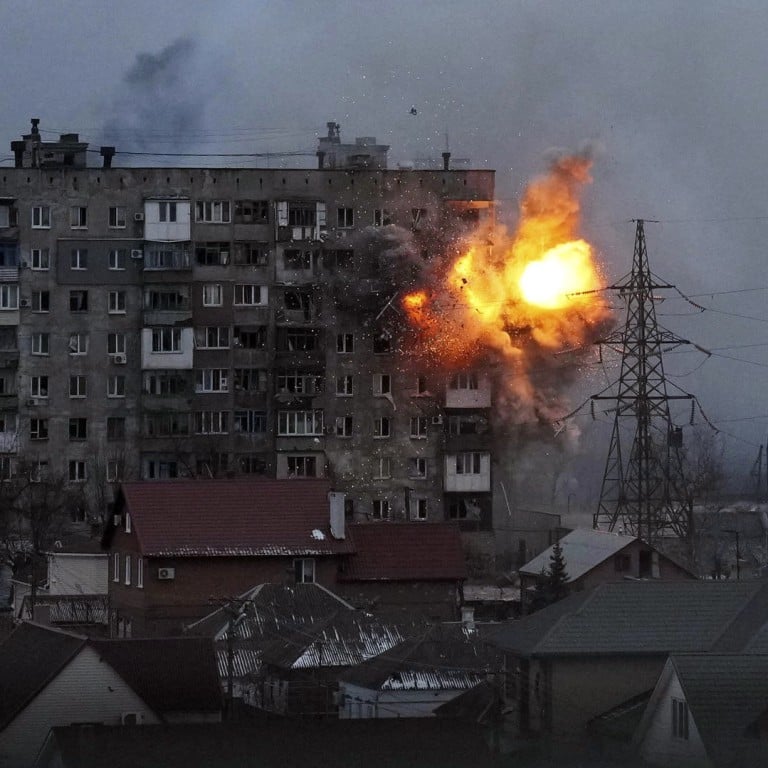The photograph depicts a dramatic explosion in a tall, multi-story residential building, likely around ten stories high, with numerous windows and small balconies. The building appears to be a dark brown color. The explosion occurs near the top floors, possibly the 6th or 7th, releasing a bright fireball of white, yellow, and red hues, enveloped by thick, almost black smoke. Additionally, debris including pieces of glass and concrete can be seen scattering from the blast. The sky in the backdrop is a dark, gloomy gray, adding to the somber and war-torn atmosphere. Adjacent to the building, there is a large power antenna or electrical tower. Below, several smaller residential houses of various colors, including reddish-brown and grayish-green, can be discerned, although the dark, cloudy skies obscure some details. The ground is dusted with snow, further contributing to the overall bleak setting.